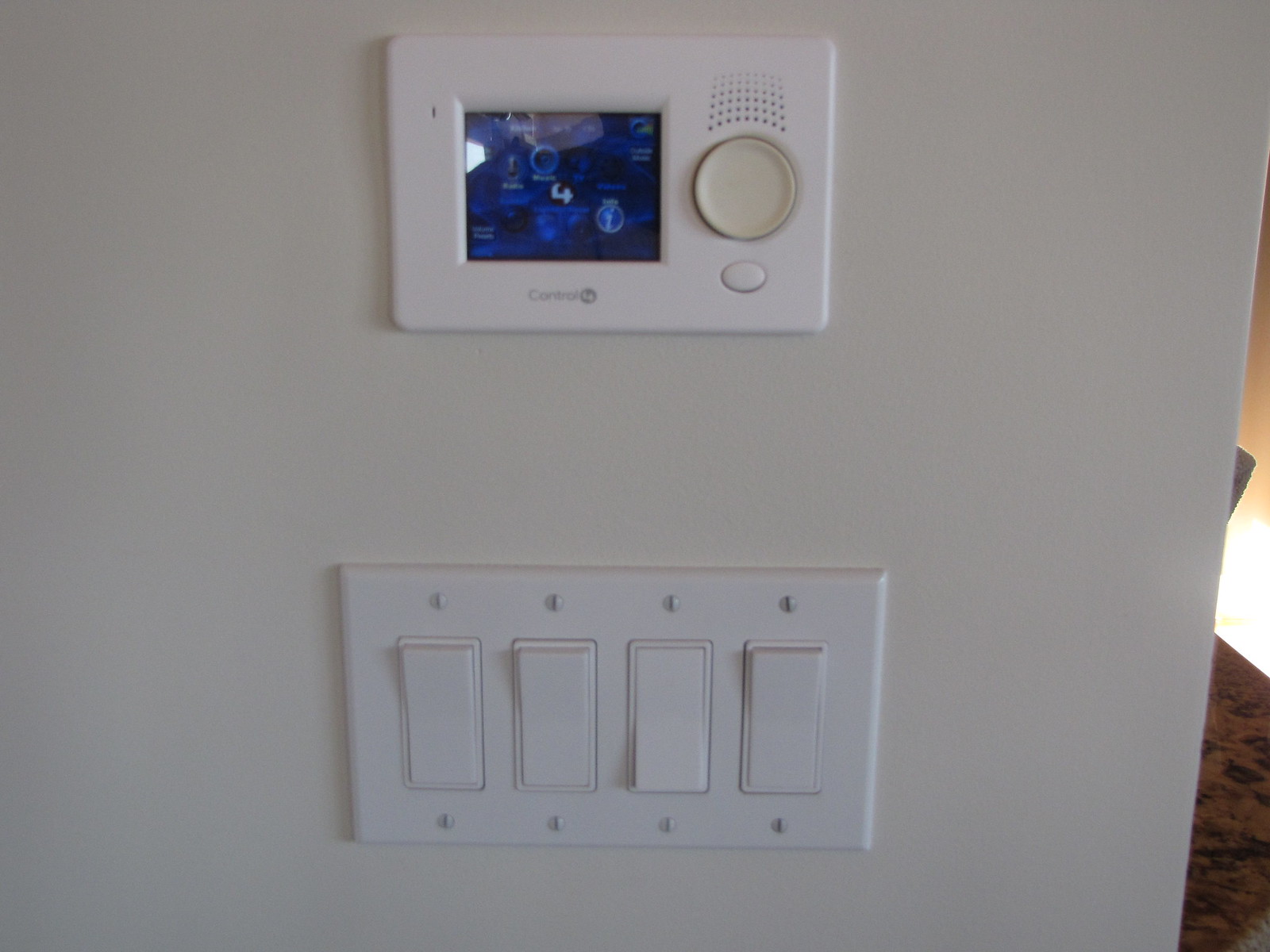The image depicts the interior of a home, featuring a pristine white wall. Mounted on the wall is a modern, white rectangular device with a circular button at the top and an oval button below it. The device appears to have small perforations, possibly indicating a speaker for voice activation. The digital screen on the device displays a blue interface with indistinct images and a partially visible label that starts with "Control."

Beside the device, there is a rectangular light switch panel, notably thicker and more modern than traditional light switches. This panel comprises four vertically aligned buttons, each secured with screws at the top and bottom, typical of a sleek, contemporary design. The first, second, and fourth buttons appear to be switched on, while the third one is off. 

Additionally, a lamp is positioned in the right-hand corner of the room, providing a cozy ambiance to the space.